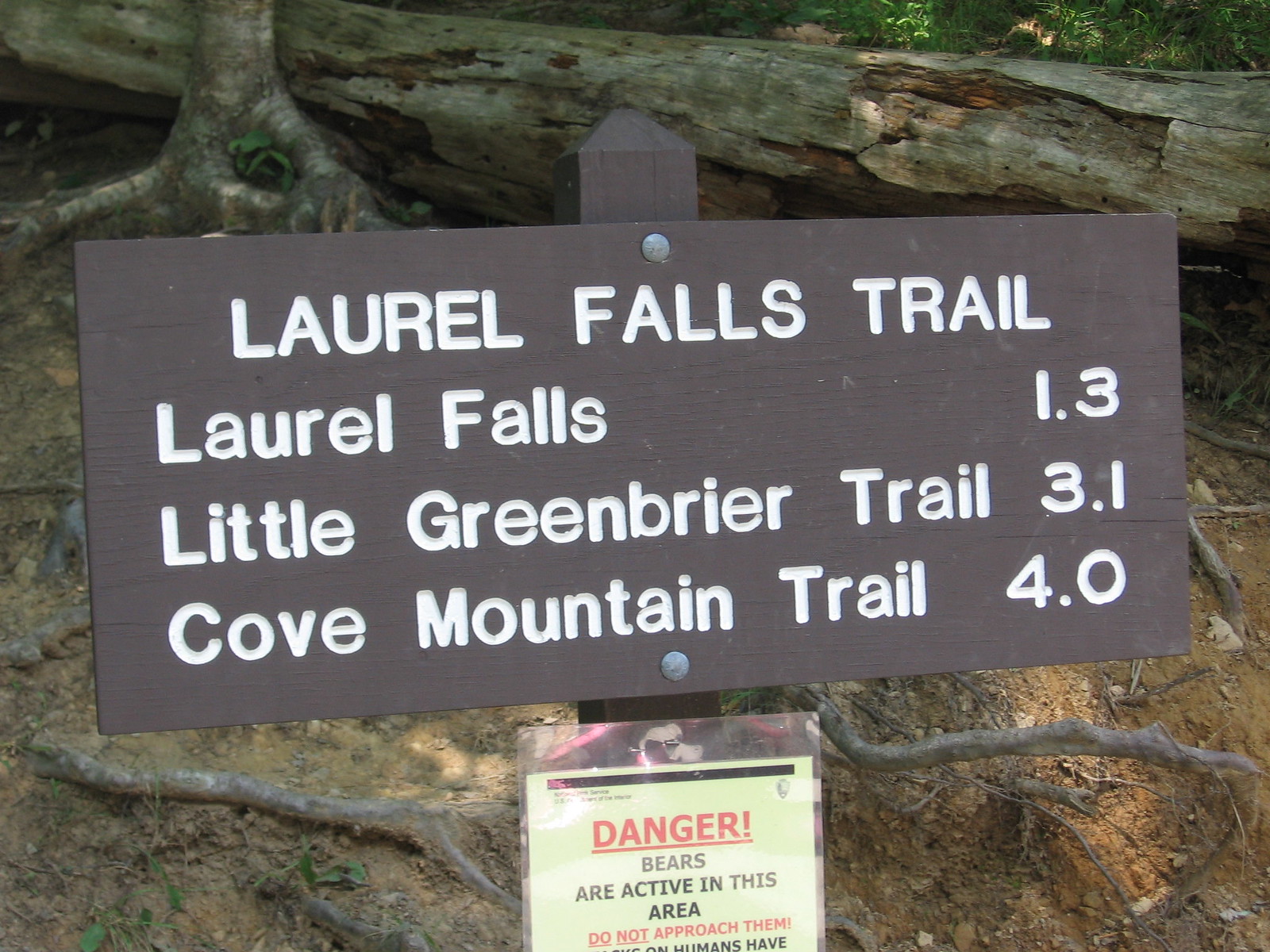In this detailed outdoor photograph, the focal point is a robust sign mounted on a wooden post. The metal sign, appearing dark gray and sturdy, clearly displays "Laurel Falls Trail" in white engraved letters. Beneath this title, it lists trail distances: "Laurel Falls 1.3," "Little Greenbriar Trail 3.1," and "Cove Mountain Trail 4.0." Below this, a laminated yellow sign carries a stark warning. In red letters, it reads "Danger," followed by a caution in black, "Bears are active in this area," and emphasized in red below, "Do not approach them." The sign is situated in a forested setting, where the background reveals a fallen tree with exposed roots, a standing tree, and dry, earthy terrain, adding context to the rugged environment.